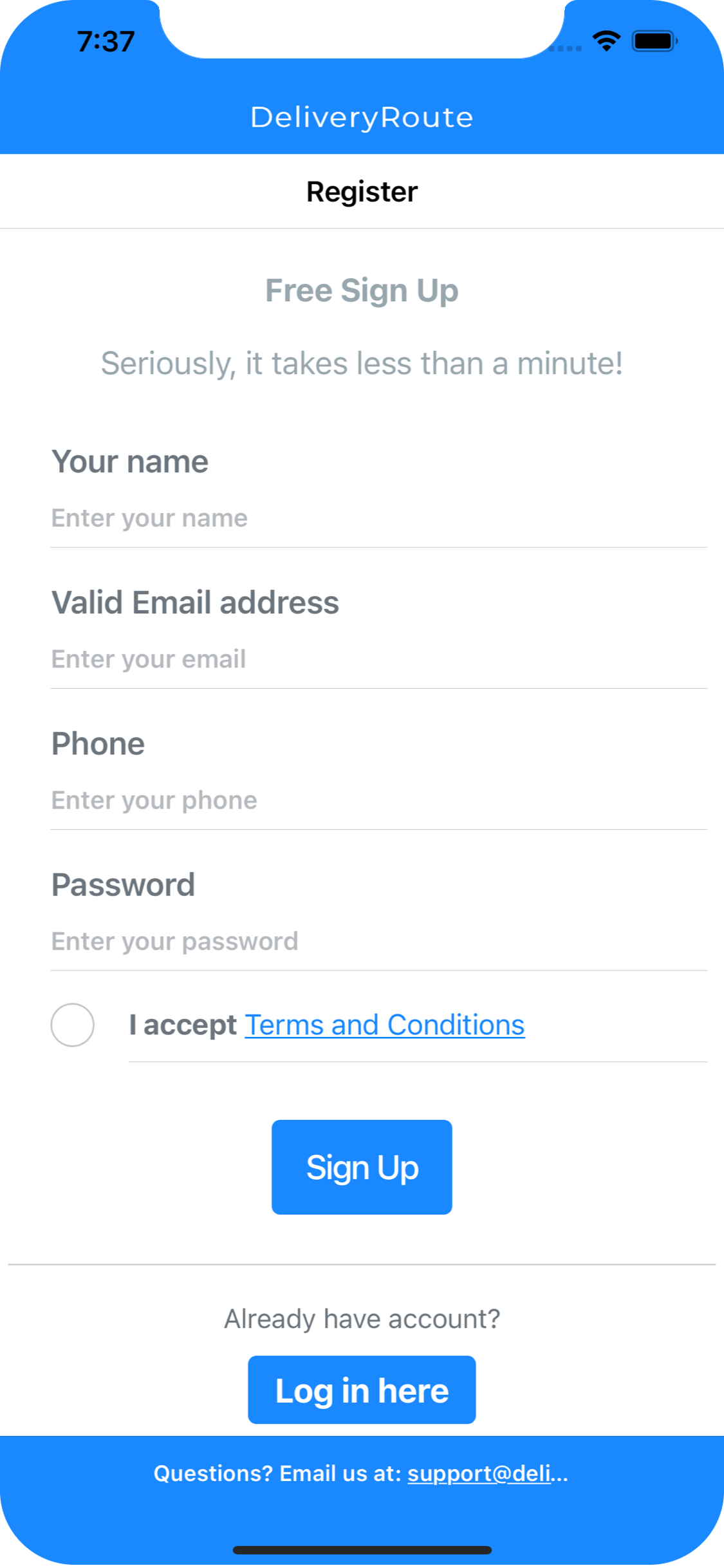The image depicts a user registration form set against a clean white background, accented with blue sections at the top and bottom. The form is not filled out, hinting at its readiness for new user input.

1. The top left corner shows the current time as 7:37.
2. Centrally positioned, there's a prominent title reading "Delivery Route," suggesting the service the form relates to.
3. Directly beneath this title, the form prompts users with "Register" followed by a dividing line before encouraging, "Free sign up. Seriously, it takes less than a minute!"
4. Below this, the form requires several pieces of user information:
   - **Name**: Next to the label "Your Name," an empty box invites users to "Enter your name."
   - **Email**: Following the label "Valid Email Address," a blank box asks users to "Enter your email."
   - **Phone**: Adjacent to the label "Phone," another box is present to "Enter your phone number."
   - **Password**: Below the label "Password," a final box awaits users to "Enter your password."
5. To comply with terms, there's a clickable circle labeled "I accept terms and conditions." The text "terms and conditions" is highlighted in blue, indicating a link.
6. For submission, a bold blue button labeled "Sign Up" stands out.
7. Beneath the sign-up button, users already registered are prompted with "Already have an account?" followed by a blue, clickable "Log In Here" button.
8. At the very bottom, a partially visible blue bar bears the text "Questions? Email us at support@deli..." (the email is cut off).

The image overall has a minimalist and user-friendly design, with blank input fields highlighting where the user information should be entered and blue elements emphasizing interactive parts of the form.